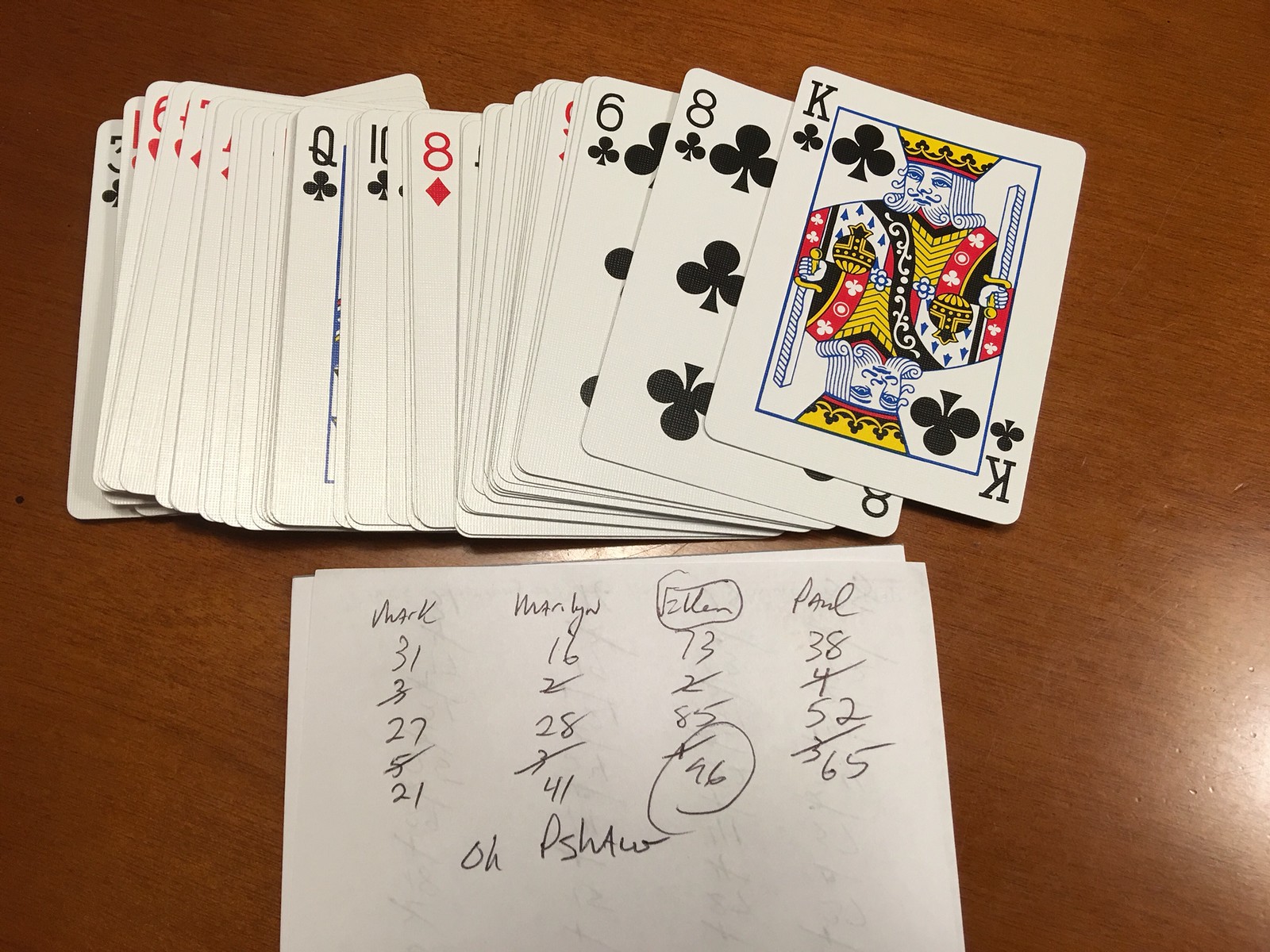The image depicts a disorganized card deck spread out on a brown wooden tabletop. Below the cards, there's a sheet of paper listing names such as Mark, Marilyn, Ellen, and Paul, along with corresponding numbers, suggesting they were keeping score for a game. The scores appear under a title, possibly "OPHSHAW" or a similar word, although the exact spelling is unclear. The scene suggests the aftermath of a casual card game, with cards and paper haphazardly arranged on the table.